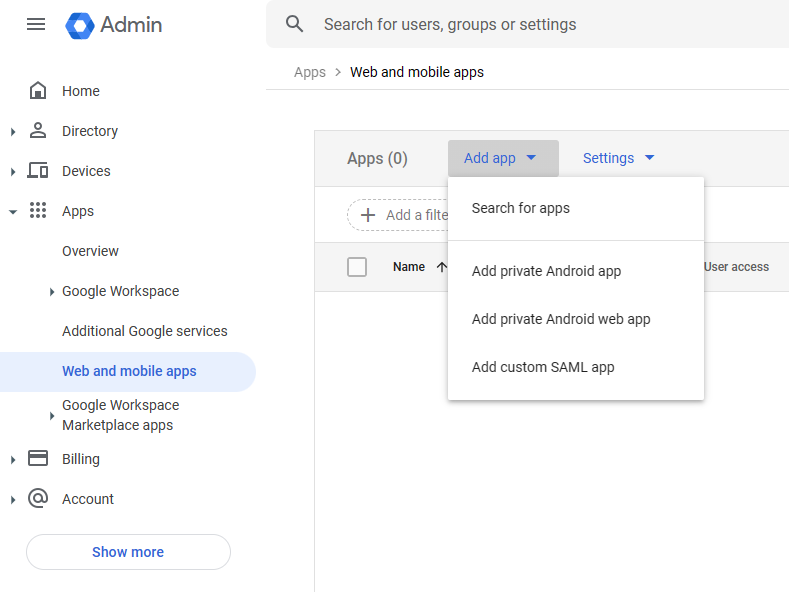The image is a screenshot taken from a website with a predominantly white background. On the left side, there is a vertical navigation panel featuring several sections and icons. The topmost part of this panel includes three horizontal gray lines, followed by a blue logo labeled "Admin" in bold, with only the letter 'A' capitalized. 

Below the 'Admin' label, the navigation items listed vertically include: 

1. A house icon alongside the text "Home."
2. A person icon labeled "Directory."
3. Icons of a laptop and a phone with the text "Devices."
4. A square formed from three dots (at the top, middle, and bottom) accompanied by the word "Apps."
5. Subsequent sections labeled "Overview," "Google Workspace," "Additional Google Services," and "Google Workspace Marketplace Apps."
6. A blue banner text stating "Web and Mobile Apps."
7. The section concludes with "Billing and Account" and a link labeled "Show More" in blue text on a white background.

On the right side of the image, there is a search bar with a gray background. Within the search bar, placeholder text reads "Search for Users, Groups, or Settings." Below the search bar, there is a heading "Apps" followed by "Web and Mobile Apps" in bold black text.

Further down, another "Apps" section appears, displaying a count of "0" apps and an option to "Add Apps" via a dropdown menu. The dropdown options include:

- Search for Apps
- Add Private App
- Add Private Android App
- Add Private Android Web App
- Add Custom SAML App

Lastly, the section labeled "Settings" follows, also featuring a dropdown menu.

This detailed layout reflects an admin interface for managing various applications and settings, streamlined for intuitive navigation and efficient use.